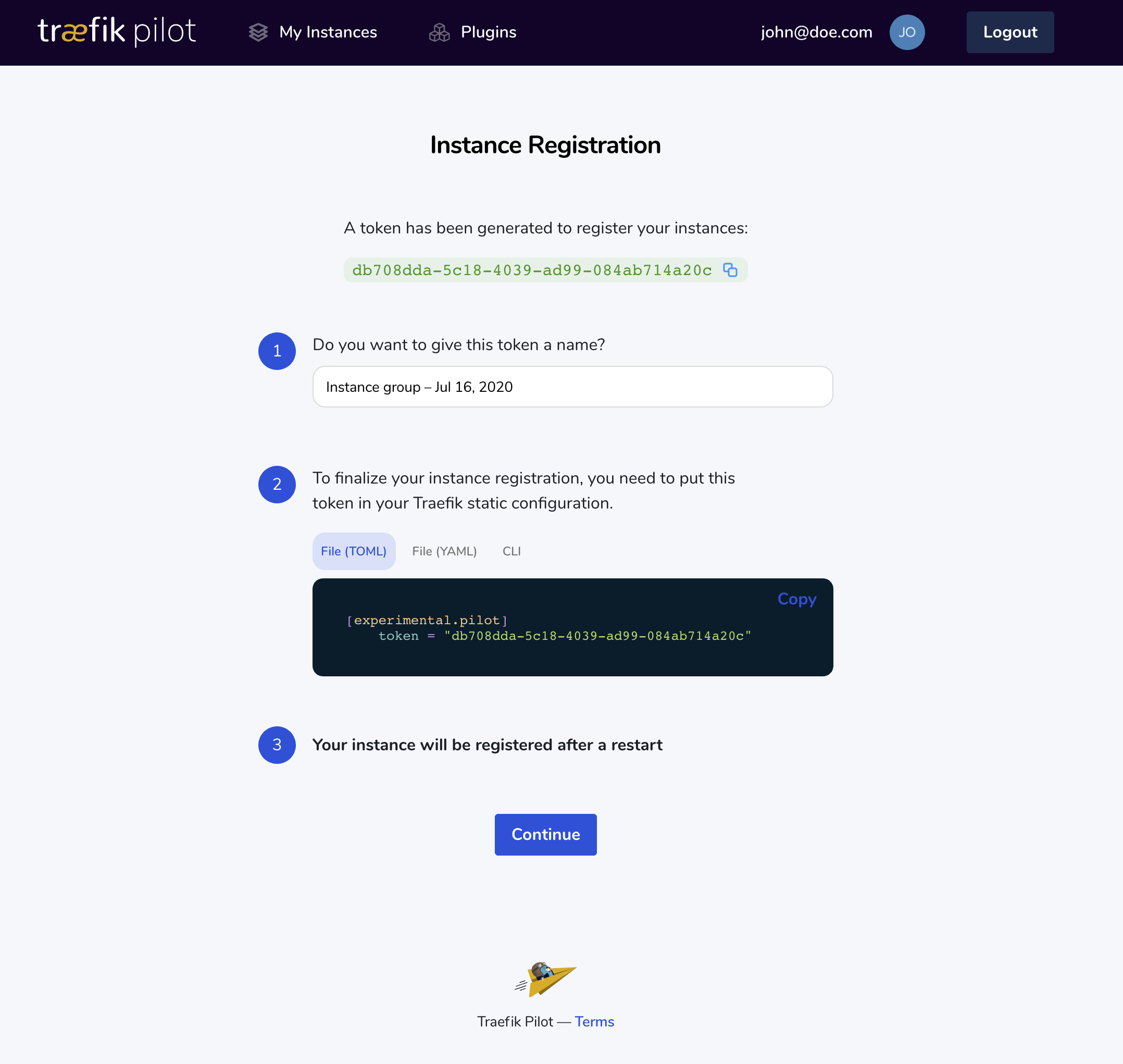The screenshot depicts the user interface of the website "Træfæik," showcasing a navigation bar at the top with links such as "My Instances" and "Plugins." The user is logged in with the placeholder email "john@doe.com," with a logout button conveniently placed nearby. The main page features a very light blue background and offers a step-by-step instance registration process.

Step 1 involves a token generation, with the interface displaying a string of randomly generated letters and numbers for the user to copy. There is an option to rename the token for better identification. Step 2 instructs users to insert this generated token into their traffic static configuration, illustrated with a helpful screenshot for guidance. Finally, Step 3 indicates that the instance will be registered upon restarting, and this process concludes with a prominent blue "Continue" button.